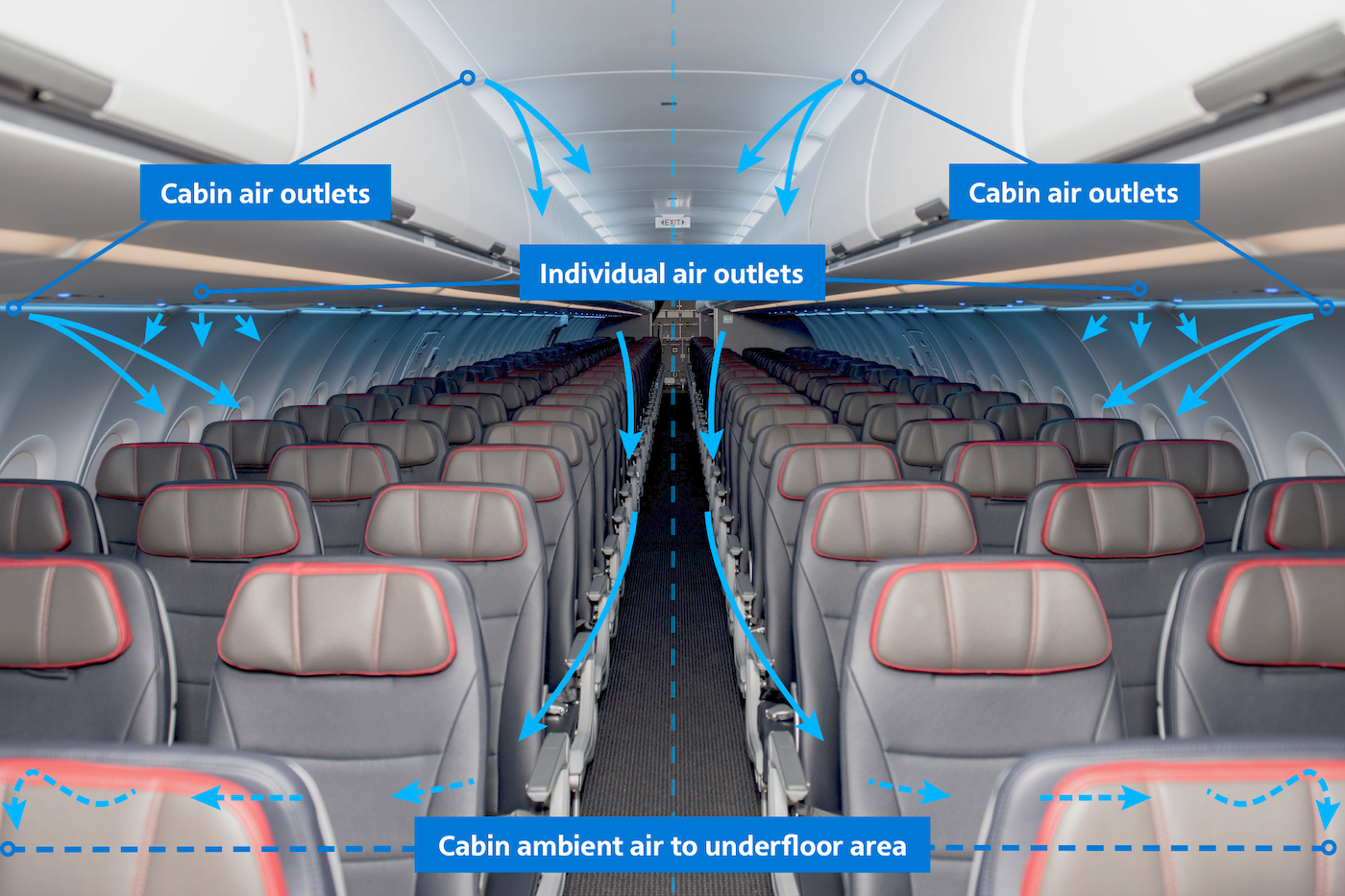This digitally rendered image illustrates the interior of an airplane cabin, focusing on air circulation dynamics. Rows of gray seats with red-outlined headrests are arranged with three seats on both the left and right sides, separated by a central aisle. Overhead bins, white with gray handles, and brightly lit cabin lights are visible. Blue arrows depict the airflow, originating from cabin air outlets at the very top, flowing downwards and through individual outlets near seat rows, and ultimately circulating to the cabin ambient air under the floor area. Text boxes label each part, providing a detailed overview of how air circulates continuously throughout the entire airplane from front to back. The image has the appearance of being part of an instructional manual, depicting the sophisticated air ventilation system designed to ensure passenger comfort.